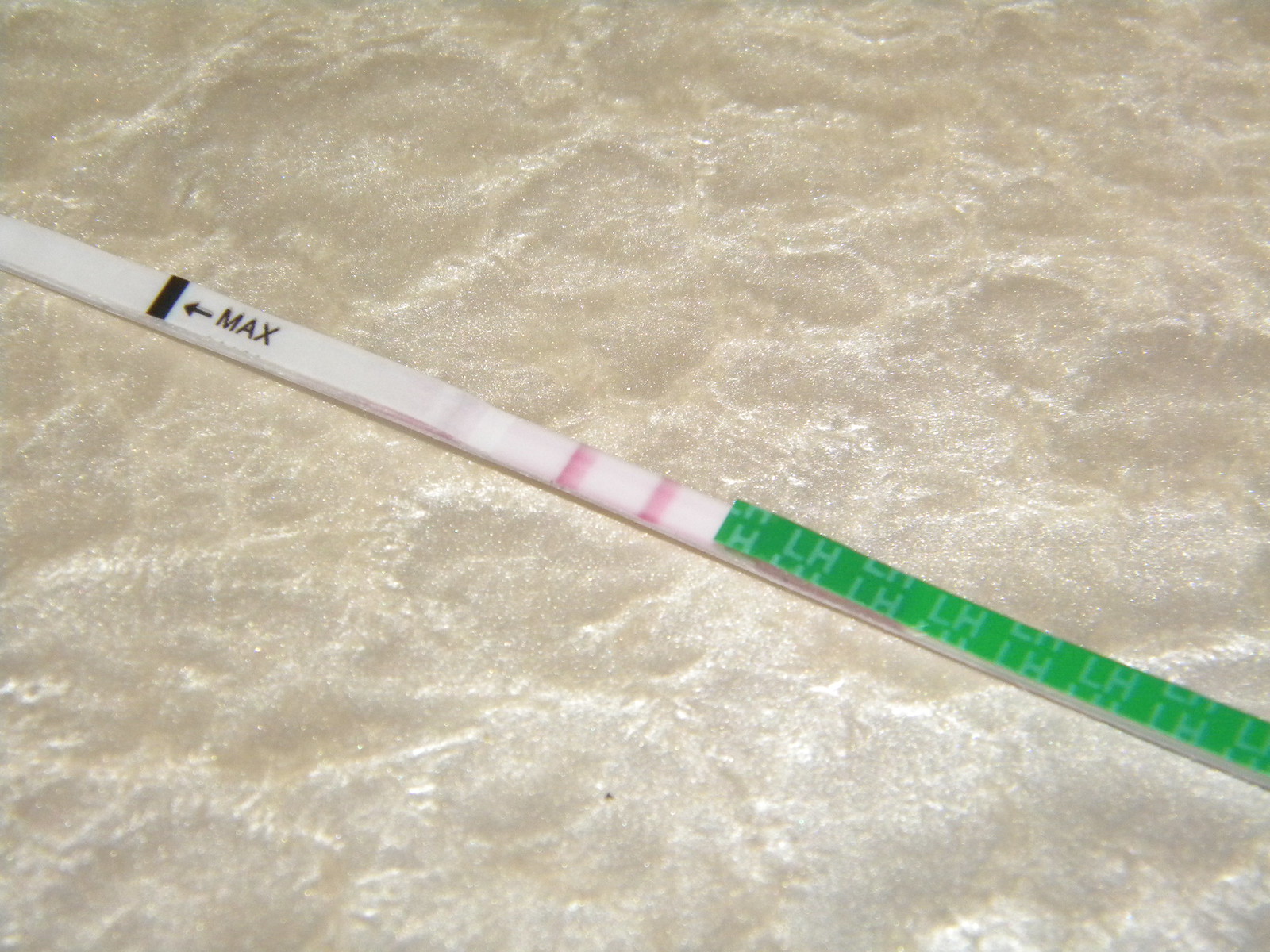The image showcases a fertility or ovulation test strip positioned diagonally on a tan, well-lit surface. The test comprises a slender, white strip with multiple colored segments. At the bottom, there is a plain white section that transitions into a black strip marked "MAX" adjacent to an arrow. Following this, there is another plain white section leading up to two spaced pink lines. Near the top, there's a green segment with the text "L-H" repeatedly printed on it. The green section appears slightly lifted, suggesting an adhesive or detachable area. The strip spans from just below the upper left-hand corner to slightly above the lower right-hand corner of the image.